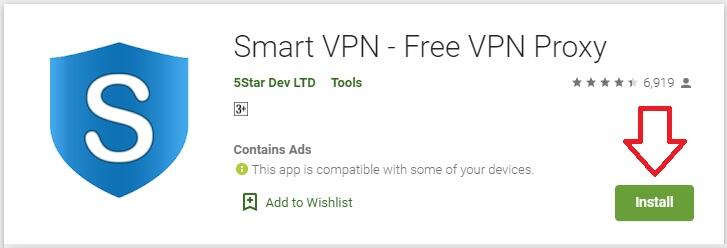In the photographic image, we see a rectangular box with a gray border. Prominently featured on the left side of the box is a blue shield graphic, which has a white "S" in its center. The top part of the box showcases the application's name, "Smart VPN - Free VPN Proxy," in the largest font with gray and black text. Below that, in green text, it reads "Five Star DDEVLTD Tools." 

To the right, there are four and a half stars displayed, indicating the app has been reviewed by 6,919 people. A profile icon is also present in this section. Written in gray text, it notes that the app "contains ads." 

Towards the bottom of the box, there's a green circular button stating that the app is "compatible with some of your devices." Additionally, there is an "Add to Wish List" tab and a red arrow pointing down towards a green "Install" button.